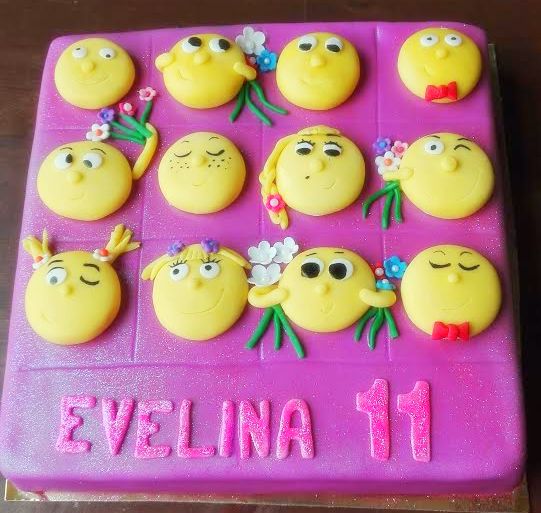This photograph features a professionally made, square birthday cake with a striking, sparkly pinkish-purple fondant as the primary color. The text at the bottom of the cake spells out "Evelina" in purple text, accompanied by the number "11," also in purple. The cake is adorned with a grid of 12 yellow circular emoji faces, arranged in three rows of four. Each emoji face showcases a unique expression, adding a playful and personal touch to the decoration. Notably, some of the faces have additional features: two are wearing red bow ties, a couple are holding flowers, and one displays a blonde braid with eyelashes. The detailed fondant work extends to these smaller decorations, all crafted from fondant in various colors. The entire cake occupies most of the image, with a slight black background transitioning to gray on the left side, accentuating the vivid colors of the cake itself.